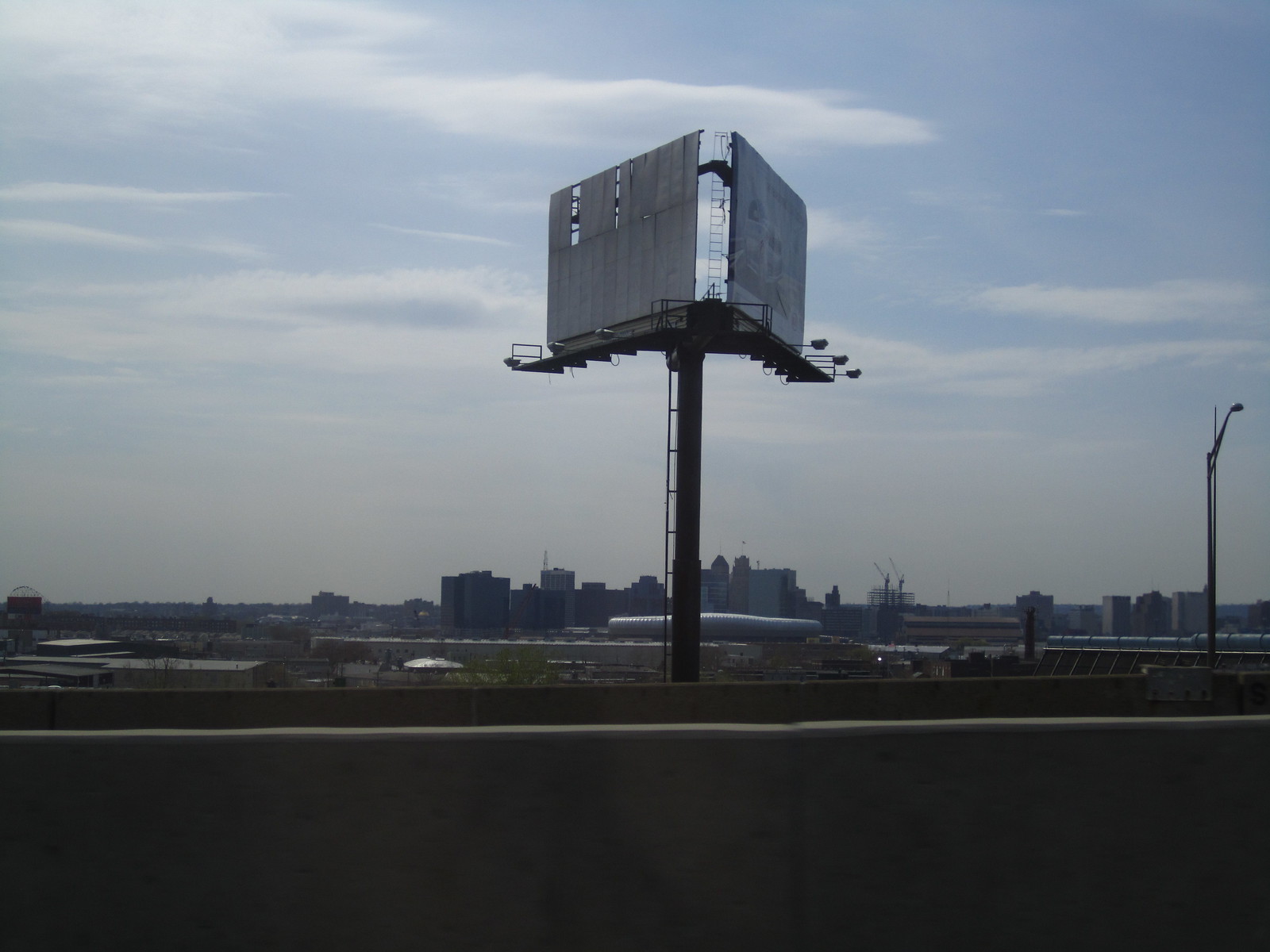The image showcases a daytime urban scene likely taken from an overpass or similar elevated vantage point. At the foreground, a tall grey concrete barrier, resembling a bridge divider, runs horizontally with a black metal pole and adjacent ladder extending vertically. Close to this, two V-shaped platforms support billboards; the left one is heavily worn and faded, suggesting prolonged exposure to the elements, while the right appears blank, possibly incomplete with sections missing. Further in the background lies an industrial area, with a potential airport dome-like structure surrounded by various smaller buildings. The cityscape, set under a clear sky with light gray and white clouds transitioning to blue, features multiple business buildings typical of a downtown district.